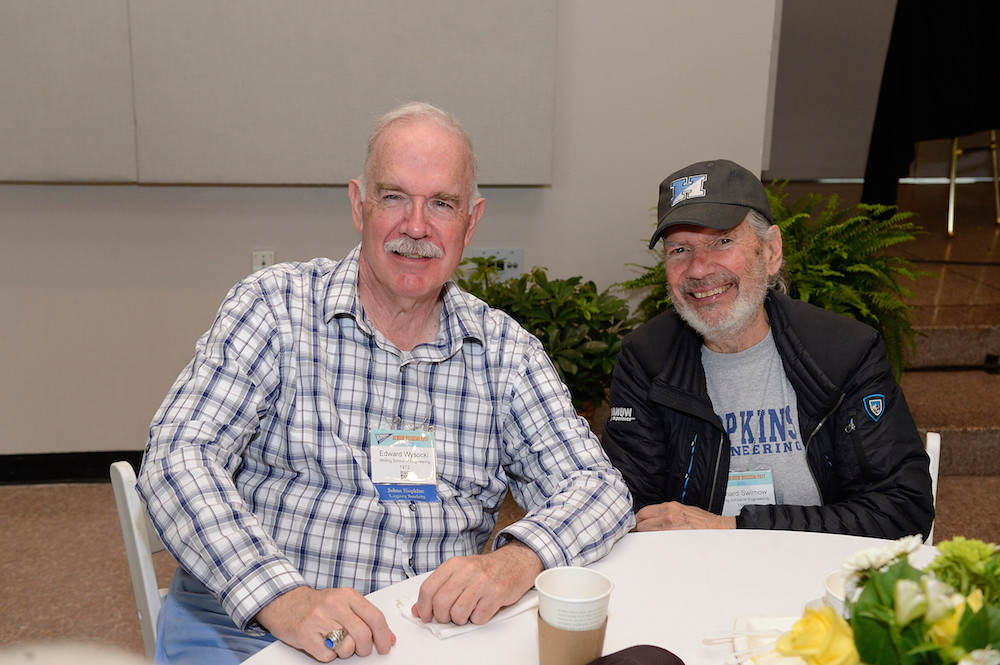In this image, two elderly men are seated at a round table covered with a white tablecloth. This table, positioned towards the bottom right corner, holds a variety of items including a bowl of white and green flowers, a white napkin, and a cup. The two men, situated at the center of the image, are outdoors, likely at a restaurant or a conference setting, indicated by the hard surface they are on and a grayish-brown building seen in the background along with some green bushes. The gentleman on the left has a graying mustache, is balding, and wears a blue and white striped, checked shirt with a placard around his neck. His blue pants match the calm palette of his attire. The second man, to his left, sports a black jacket adorned with symbols on the arms, a black cap with the letter 'H,' and a t-shirt that reads "Hopkins Engineering," also complemented by a placard. Both men are smiling warmly, creating a pleasant atmosphere in this mid-day setting. The color scheme of the image includes tan, gray, blue, light blue, green, black, and white, creating a serene, well-balanced visual.